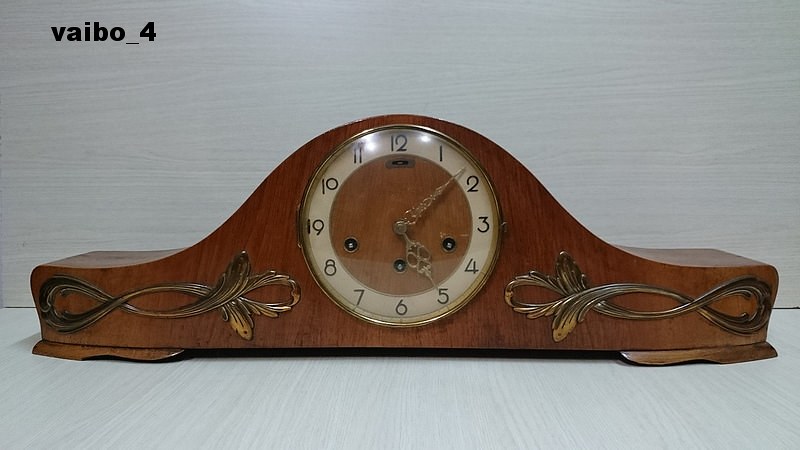This close-up photograph showcases a beautifully designed clock against a white background, prominently positioned at the center of the frame. The clock is encased in an elegant wooden frame that features a straight horizontal line at the bottom. The sides of the frame extend upward before curving inward and climaxing in a half-circle, forming a graceful arch around the clock face.

At the heart of the clock lies a striking face, encircled by a border of brushed gold. The center of the clock face is a vivid reddish-orange hue, encircled by a white strip that serves as the backdrop for the black, bolded numbers. The numbers are well-defined and arranged in a classic layout, making them easy to read.

The clock's hands are crafted from gold metal and are adorned with intricate circles and etched designs, adding a touch of elegance to the timepiece. Below the numbers 8, 6, and 4, three circles with white centers draw attention, accompanied by delicate metal leaves on each side. These leaves, resembling infinity signs with leaf tips pointing towards the clock's face, lend a sophisticated decorative touch to the overall design. The attention to detail and the harmonious blend of colors and materials make this clock a stunning focal point.